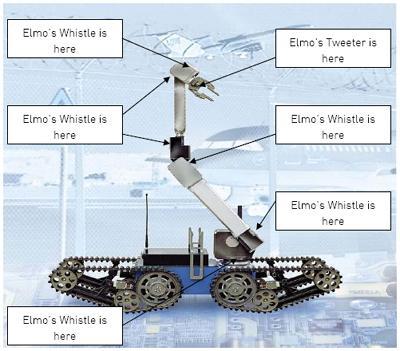The image depicts a small, child-like robotic vehicle, reminiscent of a DIY project or a Lego set. This compact robot boasts gear-like wheels and a blue base, with a main body primarily composed of silver and black elements. Its standout feature is a crane-like robotic arm extending from its body, terminating in a gray hook-like piece. The background has been altered to a pale blue, giving a light and whimsical feel, and is complemented by a series of white callout boxes outlined in black. These callouts, linked by black arrows, repetitively annotate various parts of the robot, with most labels declaring "Elmo's whistle is here" and a prominent label on the arm stating "Elmo's tweeter is here." The overall setting and labeling suggest this is a diagram, possibly instructional, aimed at illustrating different components and their functions in a playful manner.